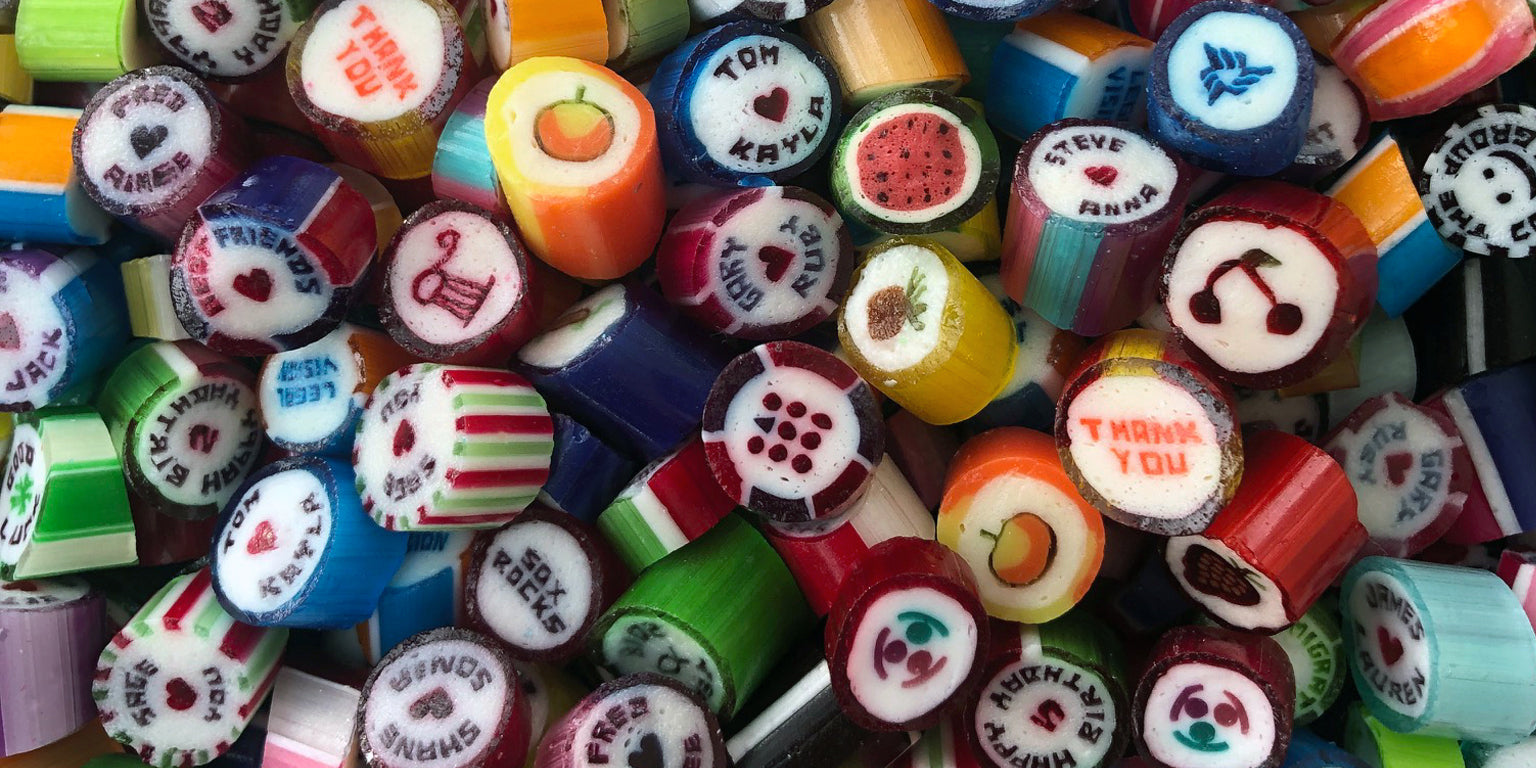This close-up image showcases an abundant assortment of vibrant hard candies, reminiscent of a nostalgic treat. Each candy is cylindrical with flat, white surfaces that feature intricate illustrations, ranging from fruity pictures and various types of insignia to heartfelt messages like "Tom loves Kayla." The sides of these candies display a spectrum of bright colors including solid hues of red, orange, and green, as well as multicolored stripes of red and green, and pink and orange. This vivid array enhances the sense of diverse fruit flavors within the mix. The candies are assembled in a disorderly pile, making it a colorful, chaotic yet delightful visual feast.